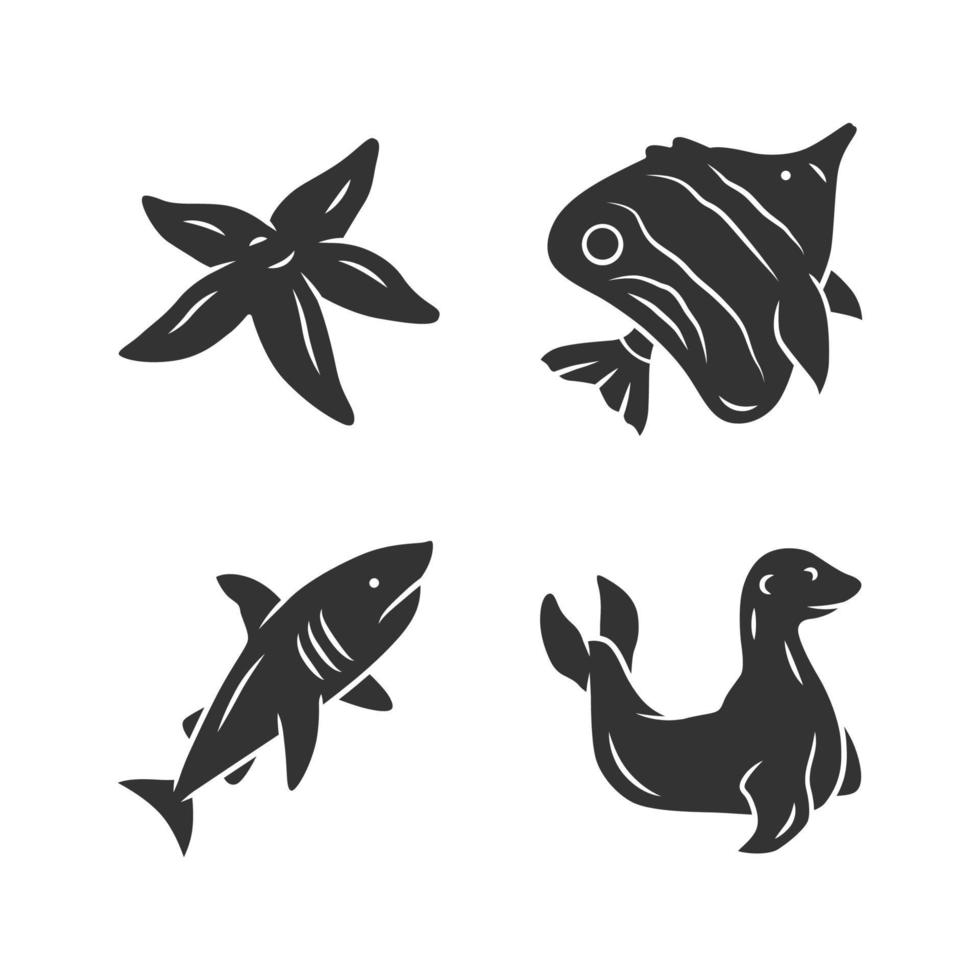This image features four stylized black-and-white illustrations, possibly serving as tattoos or stamps, arranged in a 2x2 grid against a white background. Each illustration is predominantly black with minimal white detailing to outline and define the shapes.

In the top-left corner, there's a simple, thick-lined representation of a starfish, though it could also be interpreted as a flower or a sea anemone due to its ambiguous design. The top-right corner showcases a tropical fish, likely an angelfish, with its nose pointed upward and to the right. The fish's body is mostly black, with intricate white lines adding definition and curvature, and a distinct eye marking for added realism.

The bottom-left corner features a stylized shark, characterized by a small white dot for an eye and three white gill slits. The overall posture of the shark has its nose pointing towards the upper-right corner and its tail angled downwards towards the bottom-left. Lastly, the bottom-right corner depicts a cheerful seal with its head and tail raised, rendered in the same thick black style with white accents emphasizing its joyful expression and body contours.